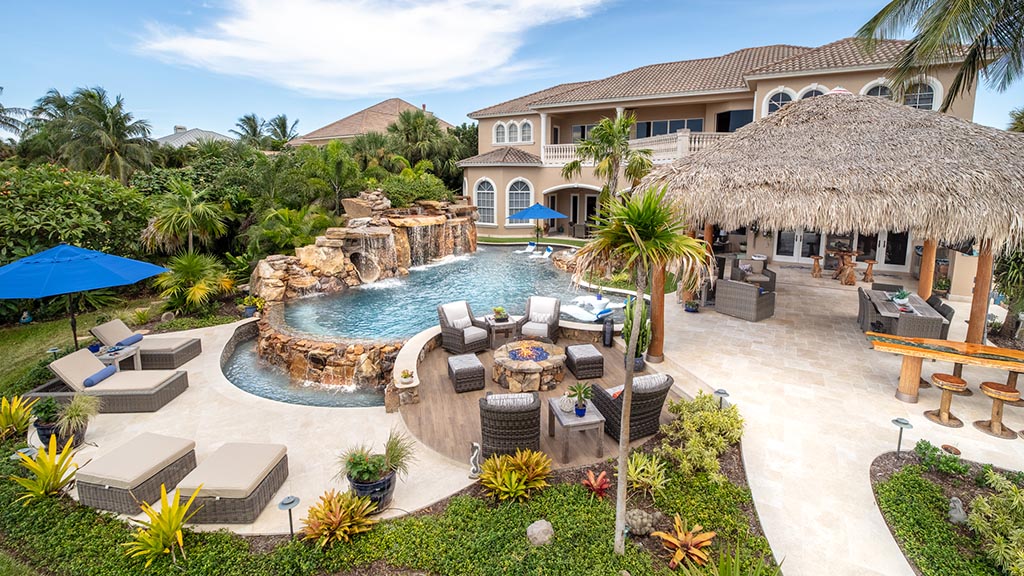The photograph captures a luxurious, semi-aerial view of a grand property, likely a mansion or resort, set in a tropical setting. Dominating the scene is a beautifully designed swimming pool encircled by an ornate rock wall featuring a cascading waterfall. The pool area is dotted with blue umbrellas and numerous lounge chairs, perfect for relaxation. Additionally, there are several designated areas for socializing, including a fire pit encircled by six seats and a thatched cabana hut with no sides, held up by wooden posts, offering a shaded table and chairs beneath.

In the background, the impressive two-story house is prominent, boasting balconies, numerous windows, and a traditional tile roof. Underneath one of the balconies is a cozy lanai section furnished with a table and chairs. The pool area also includes unique decorative elements, such as a marooned small boat on top of the rock wall, adding to the whimsical charm. The landscaping around the pool is lush, featuring shrubbery, lower grass in the lower right, and meticulously placed brown tables with accompanying barstools. A stone walkway meanders through the pool area, leading to the cabana and further enhancing the inviting ambiance of this stunning property.